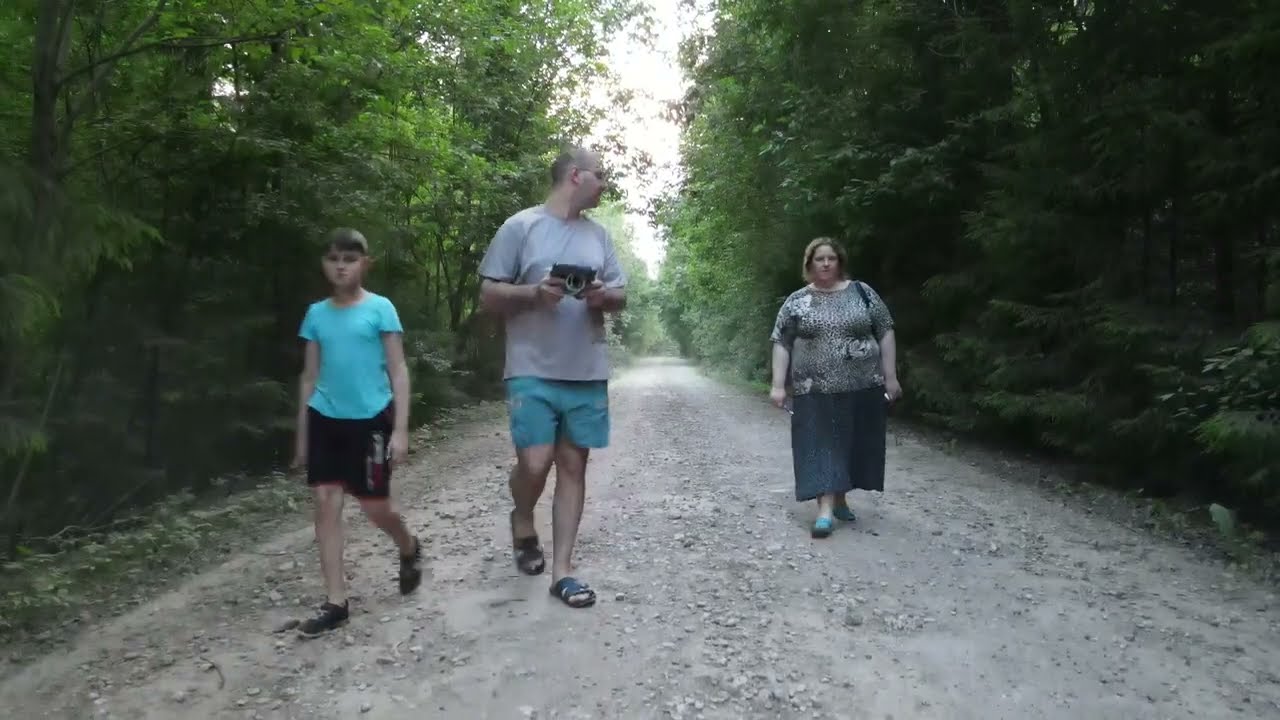In this image, three people are walking on a rocky and dirt-filled path through a lush, green wooded area. Tall trees with green foliage and brown branches line both sides of the path. The sky above is a light, whitish color that filters down through the leaves. On the left side, there is a young boy, likely around 13 years old, wearing a light blue shirt with unreadable text, black shorts, and dark-colored sneakers. In the middle, a balding man with glasses is wearing a gray t-shirt, turquoise shorts, and brown sandals. He appears to be looking back at the woman behind him while holding a dark-colored object, possibly a camera or tablet, in his hand. To the right, the woman wears a cheetah-patterned shirt with a black skirt and blue shoes. She has short blonde hair and appears to be walking slightly behind the man. The scene portrays a family taking a casual stroll through the serene and tranquil forest path.